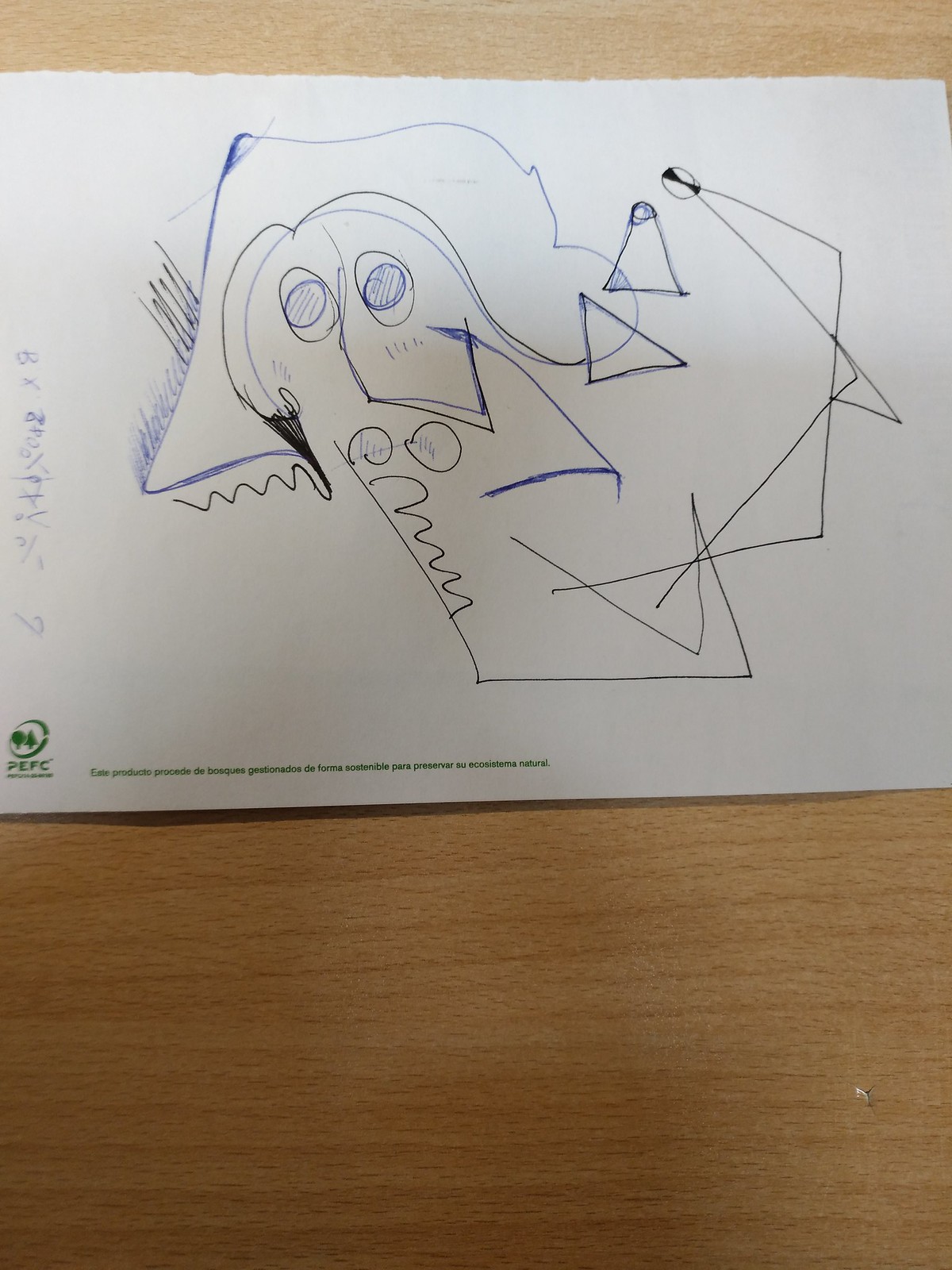A photograph showcases a sketch drawn on a sheet of paper, which features a green PEFC logo at the bottom. The logo includes a circular emblem with two trees—one with bushy leaves and the other resembling a pine tree—accompanied by some adjacent text. The sketch itself is highly abstract and reminiscent of Picasso's style. It is composed in blue and black ink and appears somewhat rushed. The drawing prominently features a large human face with a pronounced nose at the center and a pair of eyes, possibly adorned with glasses. The figure has bushy, jaw-length hair, rendered in white ink, and appears to have arms extending towards the face. Additional elements include shaded triangles scattered throughout the sketch. The sheet of paper rests on a light wood desk or table, adding to the overall composition of the photograph.